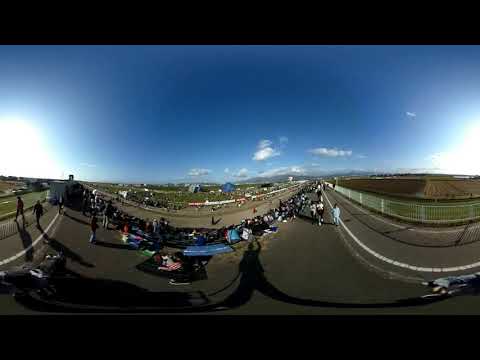This photograph captures a bustling outdoor scene on a bright and clear day. The sky is deep blue with a few clouds scattered above the horizon. The image features a walkway or bridge crowded with about 30 to 40 people, encased by fences on either side. The composition includes a unique visual effect that creates a fishbowl or 360-degree panorama, giving an illusion of the bridge extending across both sides of the image and producing two Suns at each edge, which would align if wrapped together. This effect emphasizes the curvature of the scene, making certain elements appear closer and larger. The bottom of the photograph reveals the shadow of the person taking the picture, who seems to be holding a selfie stick or a camera. The setting in the backdrop includes what appears to be grassy fields or farmland, adding a touch of nature to the otherwise busy atmosphere. The image suggests a lively gathering, possibly for an event or concert, within a vast and open natural landscape.